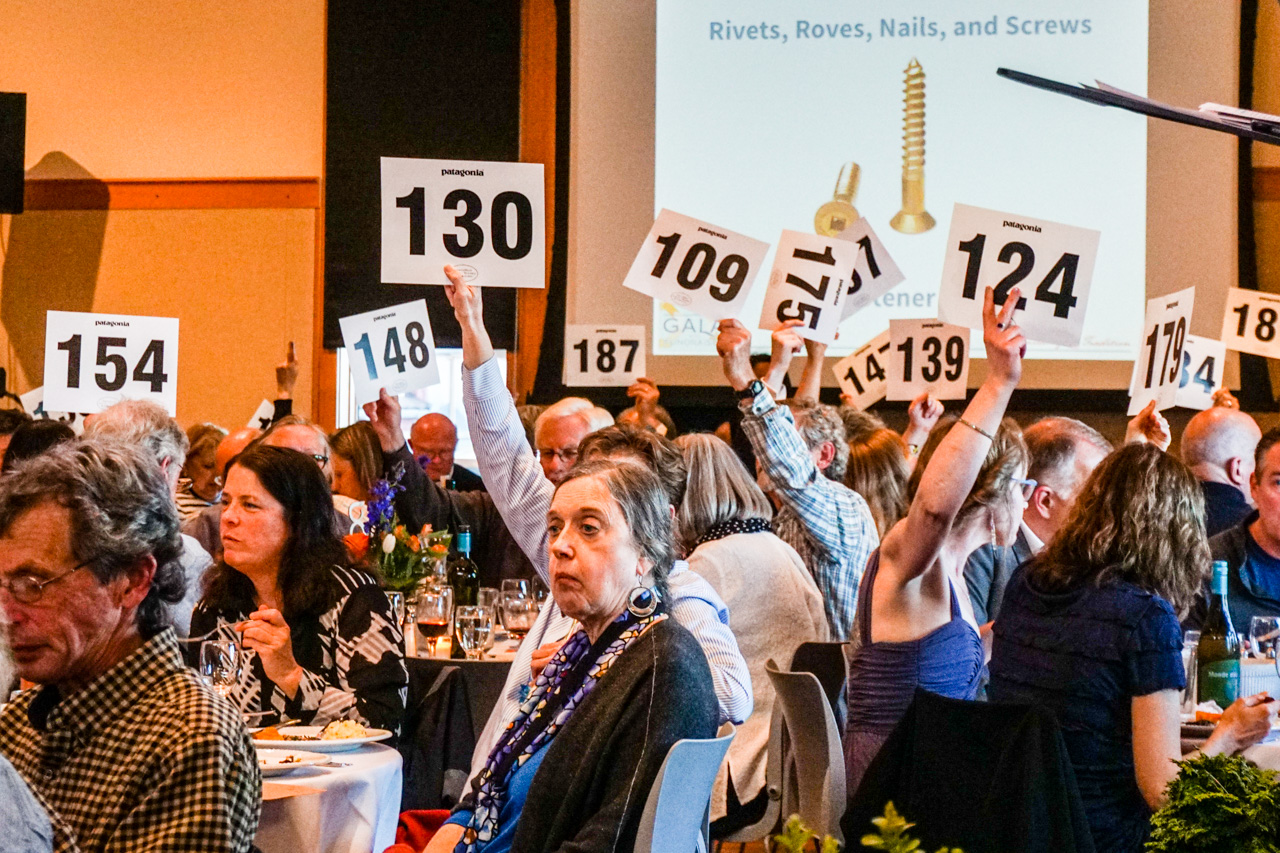A formal event is taking place in a conference room, where middle-aged to elderly attendees are seated at round tables covered with food, drinks, and elegant glassware. The participants are dressed in formal attire, including dresses, scarves, and long-sleeve collared shirts. Some attendees are holding up numbered signs, with numbers such as 124, 109, 130, 154, 148, 187, 175, 147, 139, and 179, suggesting they might be participating in a bidding activity. In the background, a projector screen displays two photos of screws with the text "rivets, roves, nails, and screws." Although the crowd is predominantly older, there is an occasional younger person present.